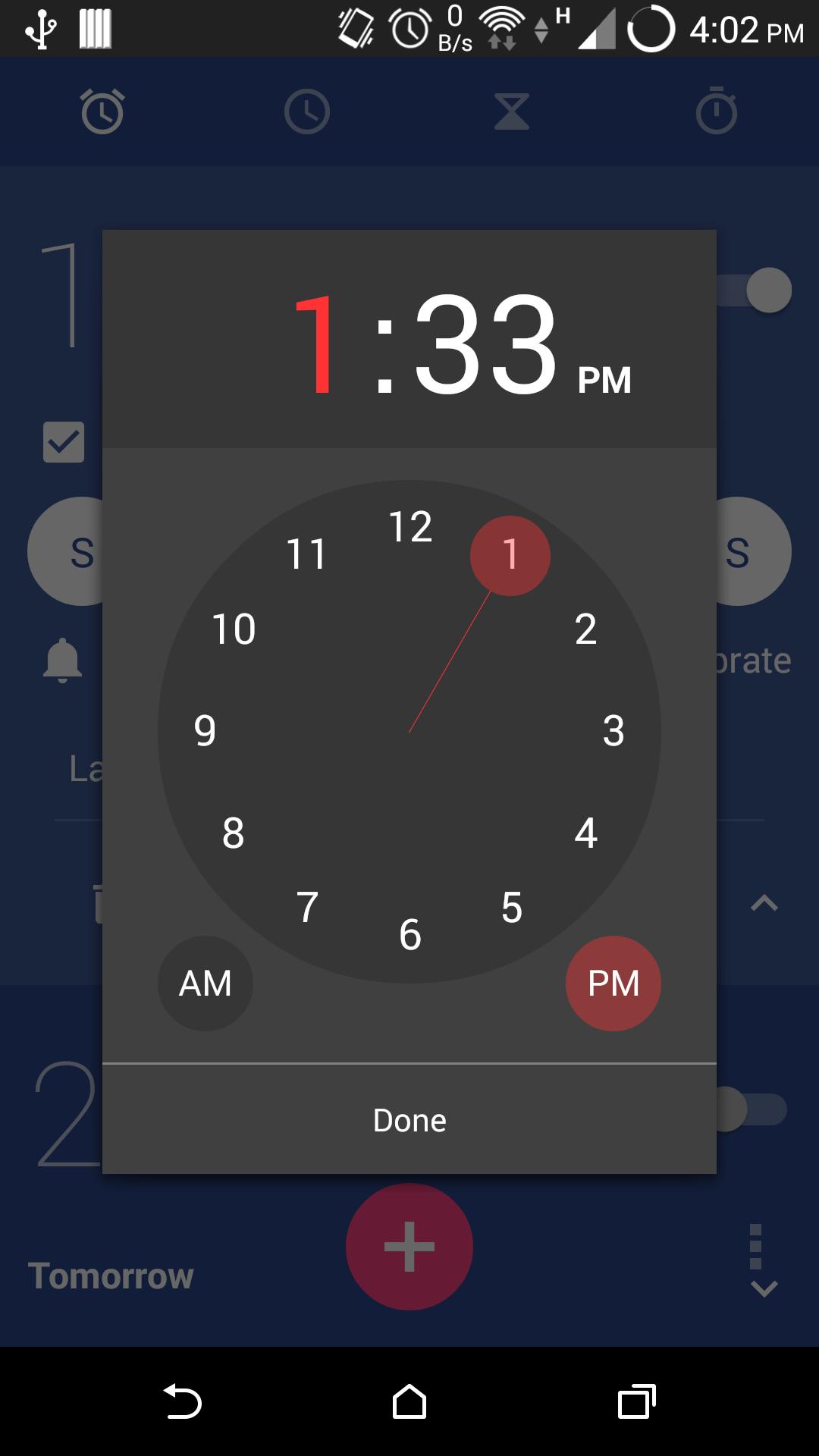This image is a screenshot of an Android mobile device's clock app at 4:02 PM. In the top right corner, there's a digital clock reading "4:02 PM". Next to the time, there is an icon of a circle, partially filled, indicating that a segment equivalent to 15 minutes is grayed out, specifically positioned at the 9 o'clock and 12 o'clock mark.

The signal strength indicator displays half of its full capacity, and beneath it, there’s an icon representing two overlapping triangles with an "H", indicating an HSPA (High-Speed Packet Access) connection. The internet connection status shows "0 B/s." Below this, a clock icon, presumably for an alarm, is present, alongside a phone icon with vibration lines, signifying the device is set to vibrate mode.

On the far left of the status bar, there are two additional icons. The first is a connection option, possibly representing a USB connection, and next to it, there are four vertical bars, representing a feature or status not specified.

The main interface is a blue background displaying options for "Clock," "Alarm," "Stopwatch," and "Timer." At the center of the screen, the user is in the process of setting up an alarm, currently set to 1:33 PM. Beneath the clock setting, there are toggle options for "AM" or "PM," allowing the user to specify the time of day for the alarm.